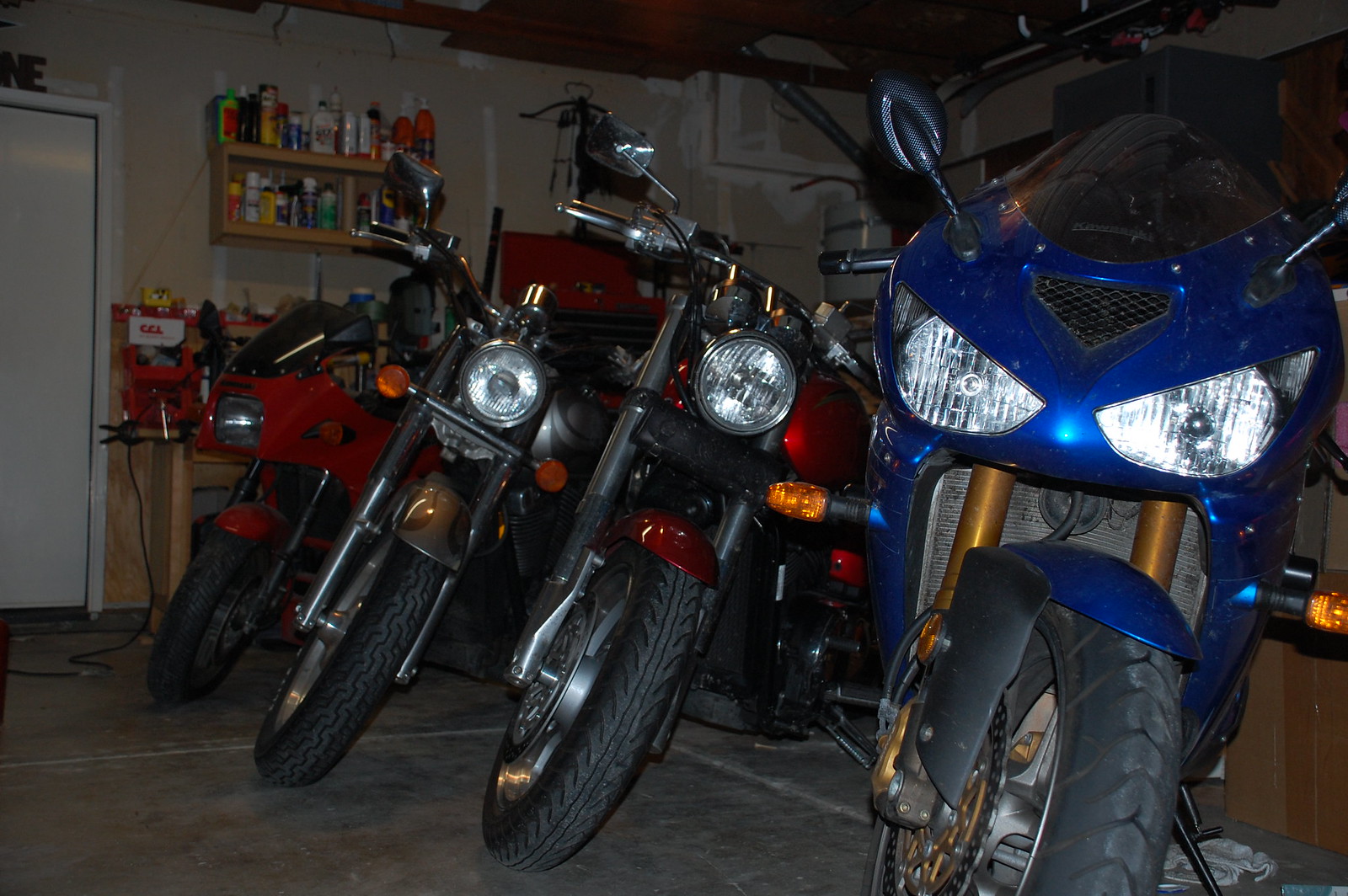This is a detailed color photograph of a cluttered garage interior, featuring four motorcycles as the main subjects. The lighting is low, casting a dark ambiance over the scene. In the background, the garage walls are unfinished with patches of grayish plaster and unpainted drywall. 

On the left side of the image is a lighter grey door marked with the letters "N" and "E." Shelves laden with various bottles and cans, likely for car maintenance or DIY projects, extend along the back wall. There's also a noticeable hot water heater and a garage door mechanism adding to the clutter.

The motorcycles are lined up from left to right. The first two are red, with the second one being a bit smaller and having a black windshield. The third motorcycle, closer to the viewer, is mostly concealed but seems to have an orange or grey tint. The fourth motorcycle, prominently in the foreground, is a shiny blue with distinctive dual headlights resembling an alien or bee face, accented by a blue hubcap and orange bars underneath. The overall floor appears dark and possibly tiled.

Additionally, a small red scooter peeks out from the corner, completing the array of motorbikes. A wooden object, perhaps a cupboard, is visible just beyond the blue motorcycle on the right side, emphasizing the utilitarian nature of the space.